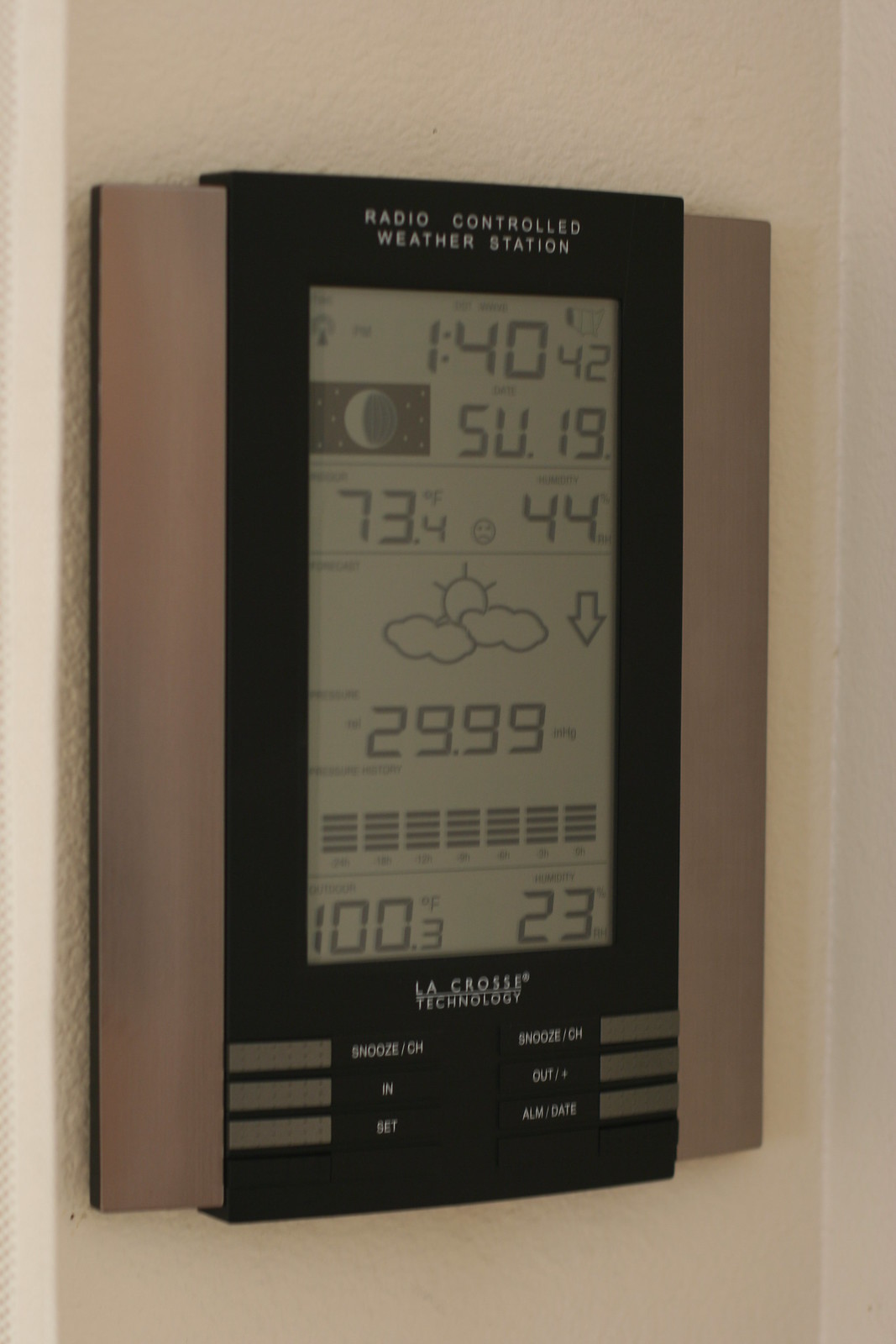In this image, a sophisticated digital weather information station is mounted on a light yellow wall. This multifunctional device, made by La Crosse Technology, serves not only as a thermometer but also as a comprehensive weather station. The display indicates the time as 1:40:42 PM on a Sunday. The current temperature is shown as 73.4 degrees Fahrenheit, with an additional reading of 44 degrees Celsius, and the weather condition is partly sunny. The barometric pressure stands at 29.99 inHg.

Additionally, the station provides a seven-day week display, from Sunday through Saturday, indicated by bars. The bottom panel, although partly obscured by the small font size, appears to show a reading of 100.3, the significance of which is unclear. The outer frame of the unit is black, and the lighting in the room casts noticeable shadows to the right of the device, suggesting a light source to the left. The lower section of the station offers buttons for setting an alarm, snooze, and outside temperature, along with the date setting. Overall, this detailed weather station is a central hub for various meteorological data and timekeeping.